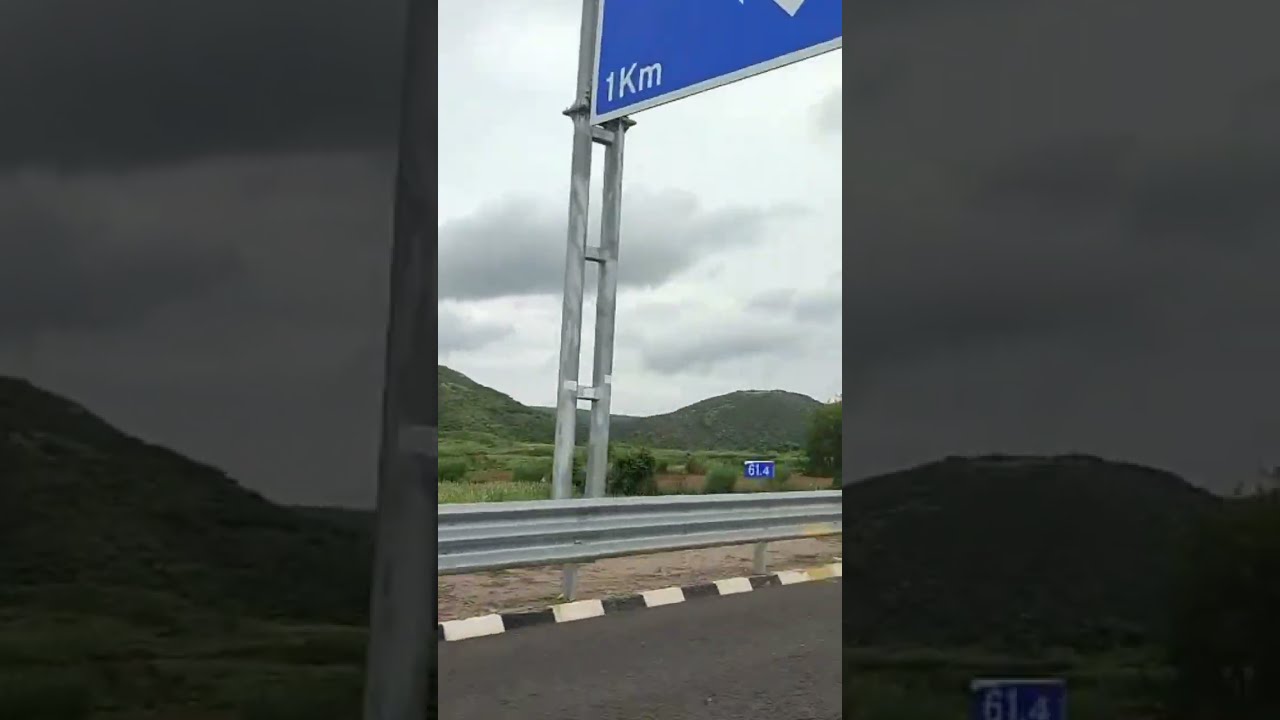The image is a rectangular photograph, layered with a narrower photograph running vertically through the center. The larger, muted background features an overcast sky with dense, gray clouds above a hilly, tree-dotted landscape. The central strip, depicting similar scenery from a further distance, emphasizes a roadside scene with detailed elements:

In the foreground, pieces of a blacktop road are visible along with a silvery guardrail. The guardrail, likely made of aluminum, runs alongside a shoulder barrier painted in white and black stripes. This strip also includes part of a blue highway sign mounted on dual metal poles extending about 20 feet high. The sign displays a "1 KM" marking, suggesting a European location, and a smaller sign denoting "61.4". A portion of the sign's metal frame is visible, situated amidst shrubbery and dirt beneath the guardrail. In the background, the same natural elements reappear with expansive hills and various greenery, all under the cloudy, glary sky. The entire composition showcases a layered, semi-monochromatic view of a European roadside and landscape, bordered by enlarged, grayed-out elements of the image.